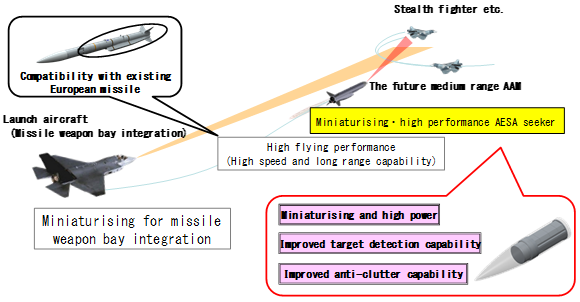The infographic in landscape orientation features a combination of illustration and typography on a white background. At the top left, there's an illustration of a missile with a detailed view, accompanied by a conversation balloon that highlights "compatible with existing European missile." Below this detail, there is another emphasis on "launch aircraft missile weapon bay integration."

Directly below, a fighter jet points towards the top right corner, emphasizing "miniaturizing for missile weapon bay integration" in a text box. The right side of the image showcases three interacting fighter jets underlined by the text "stealth fighter, etc." Just below this, another horizontal text box labels the "future medium-range AAM."

Circling downwards from here, the infographic further explains "miniaturizing high-performance AESA seeker" along with descriptions such as "high flying performance, high speed and long range capability." Another line of text notes "miniaturizing and higher power" which improves "target detection capability" and "anti-clutter capability."

The whole illustration style blends graphics of missiles and jets with various annotation bubbles and text boxes, enhancing the detailed depiction and technological specifications.